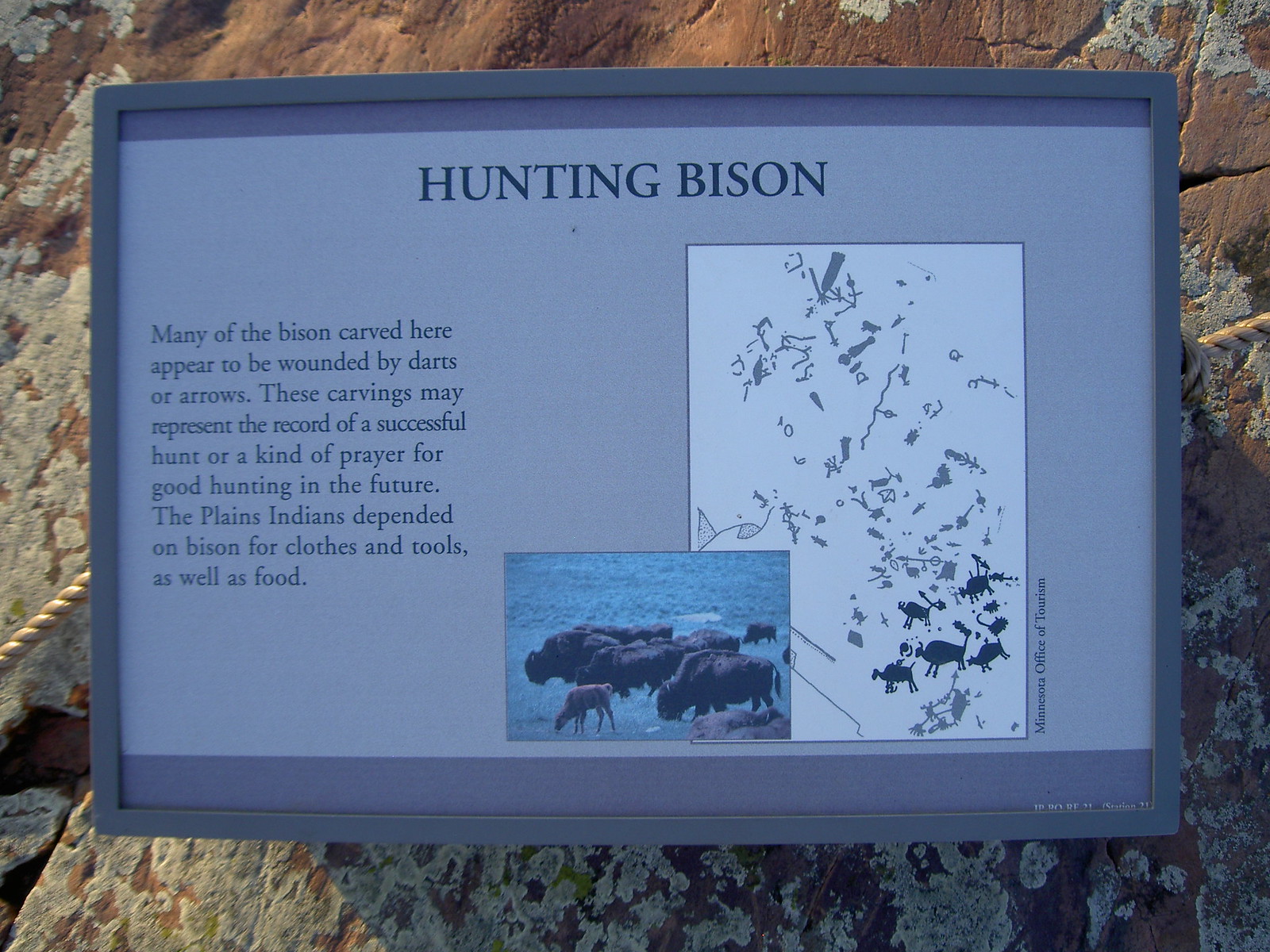The image depicts a detailed historical plaque centered and framed in various hues of blue, light purple, and gray. The plaque's headline, "Hunting Bison," is prominently displayed at the top in all capital letters. Below this headline, the plaque features a descriptive text in black lettering, explaining how many of the bison carvings shown appear wounded by darts or arrows. This suggests the carvings could symbolize a record of a successful hunt or a prayer for good hunting. The text highlights the importance of bison to the Plains Indians for their clothes, tools, and food. 

In the bottom portion of the plaque, a small horizontal photograph features bison drinking from a river, rendered with a bluish tint. To the right of this photograph is a larger, vertically positioned black-and-gray depiction of older, hand-drawn bison carvings on a white background. The plaque is affixed to a brown and white mottled stone wall, with a bit of rope visible on the far left. The Minnesota Office of Tourism is also mentioned. The overall scene blends rich cultural history with vivid imagery, framed within the rustic texture of the stone backdrop.